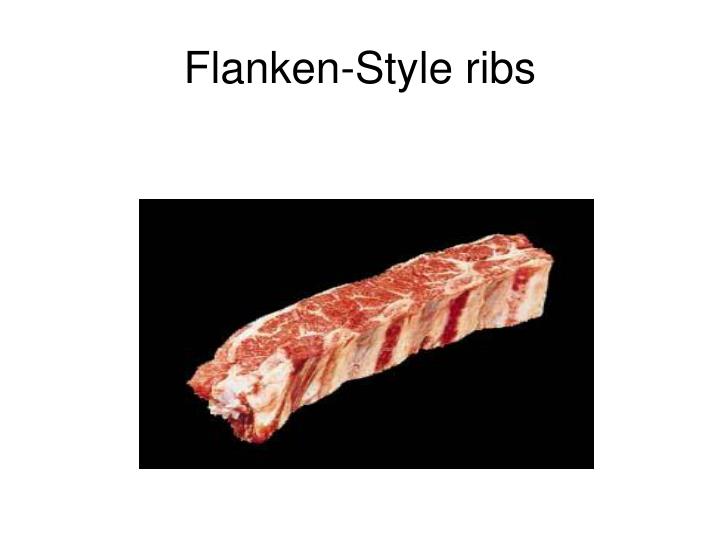The image features a raw, uncooked, flanken-style rib displayed prominently on a black rectangular background towards the bottom center of the square-shaped frame. The rib is characterized by a rich red color, interspersed with white marbling and fat, and some visible bone at the edges. Above the meat, the top half of the image has a white background with black text reading "Flanken-Style Ribs" in a simple font, with the 'F' and 'S' in uppercase. The rib, appearing to be about an inch thick, is placed diagonally from the bottom left to the top right within the black rectangle, showcasing its high-quality marbling and appealing texture. The overall image suggests a professional presentation, possibly for a website selling premium meats.